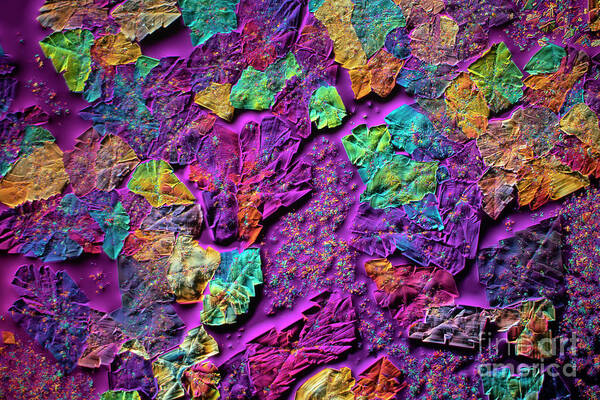This image showcases a detailed piece of abstract artwork with a strong, surreal presence. The artwork predominantly features a bright, pinkish-purple background that lends a highlighted effect, creating a vivid canvas. Emerging from this background are textured, three-dimensional projections that resemble leaves, rock faces, and possible fossils. These elements are rendered in an array of unconventional, vibrant colors including shades of brown, red, neon blue, neon green, orange, yellow, and pink. The surface of the artwork is richly textured, giving it a bumpy and rough quality that adds to its three-dimensional feel. The image, rectangular in shape, measures approximately four to five inches wide and three inches high. In the bottom right corner, a watermark in light gray, reading "Fine Art America," is visible, denoting the source of this intricate and colorful piece.